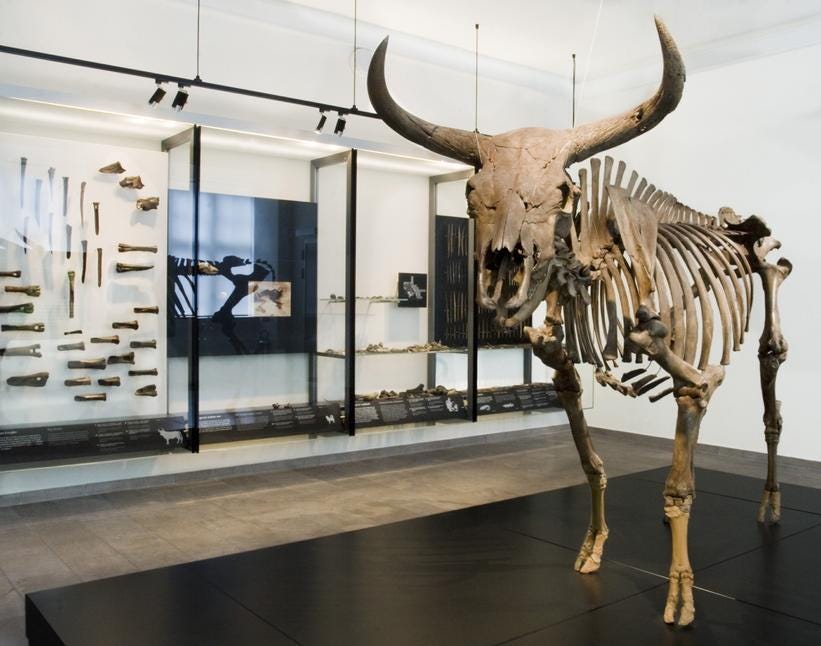This is a detailed photograph of a museum interior, likely an archaeology museum. The main subject on the right side of the image is an impressive light brown skeleton of a large horned animal, possibly a bull, bison, or ox, meticulously reconstructed and standing upright on a modern black display platform without any glass enclosure. The animal's head features prominent, curved horns that project outward.

In the background, on a white wall to the left, there are smaller singular bones and bone fragments exhibited in glass display cases, arranged neatly on small shelves. Some bones are attached directly to the wall, with spotlights beaming down from an overhead black bar suspended by silver strings. This lighting accentuates the bones against both white and black backdrops.

The museum floor consists of brown and white tiles, and the dark brown display platform contrasts with the lighter surrounding floor. Various other objects are visible but blurred, indicating additional exhibits further in the background. The walls are predominantly white, enhancing the visibility of the displayed artifacts.